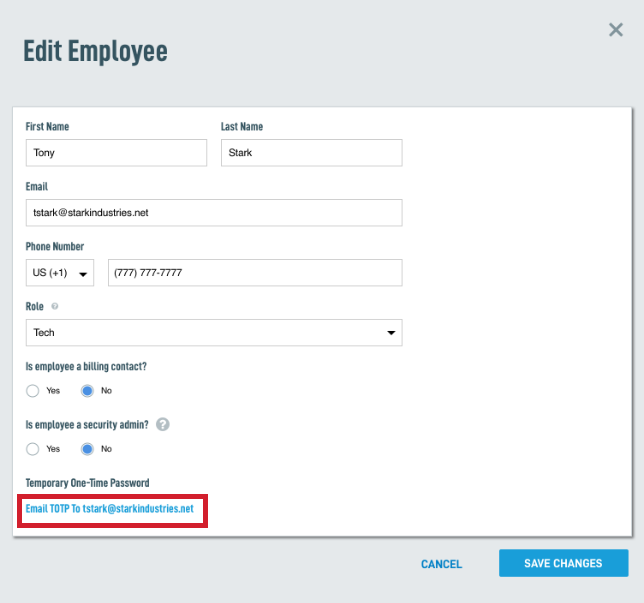Screenshot of a web form entitled "Edit Employee" displayed at the top in blue or gray font. Below the title, in a white rectangular field, there are several sections for entering an employee's information. 

The top row contains fields labeled "First Name" and "Last Name" with corresponding values entered as "Tony" and "Stark." Adjacent to these fields is an "Email" field filled with "TStark@StarkIndustries.net."

Further down, a "Phone Number" section includes a country code selector set to "USA (+1)" and a phone number field populated with "777-777-7777" representing a standardized placeholder format.

The next field, labeled "Role," has the value "Tech." Beneath this field are radio buttons for "Is Employee a Billing Contact?" with options for "Yes" and "No." The "No" option is selected.

Another set of radio buttons asks "Is Employee a Security Admin?" with the "No" option selected. 

A section for "Temporary One-Time Password" follows, highlighted with a thick rectangular outline around the field containing "TStark@StarkIndustries.net," indicating the temporary password will be sent to this email.

At the lower right corner of the form are buttons labeled "Cancel" and "Save Changes" allowing the user to discard or save the information entered.